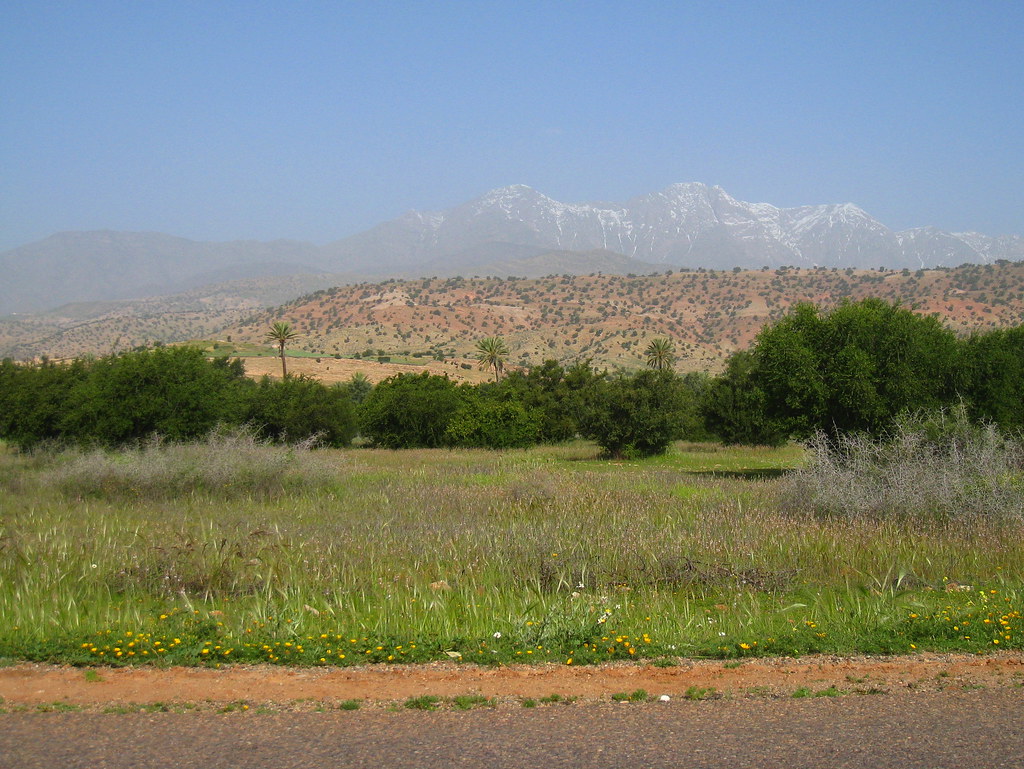The photograph captures a picturesque landscape scene in a subtropical area. In the foreground, a gravel road horizontally stretches across the frame, accompanied by yellow dandelions. Behind the road lies a thin strip of beige dirt transitioning into a lush field of green grasses dotted with a few daisies and low-lying shrubs. The verdant expanse leads to a row of dark green, short trees, including some fruit trees, with a few palm trees visible in the distance. Further back, the terrain gradually rises into a reddish dirt hillside, sparsely covered with green trees. Dominating the distant background is a majestic mountain range characterized by its sandstone appearance, capped with patches of snow. The entire scene is enveloped under a slightly foggy blue sky, adding a sense of depth and realism to the idyllic setting.